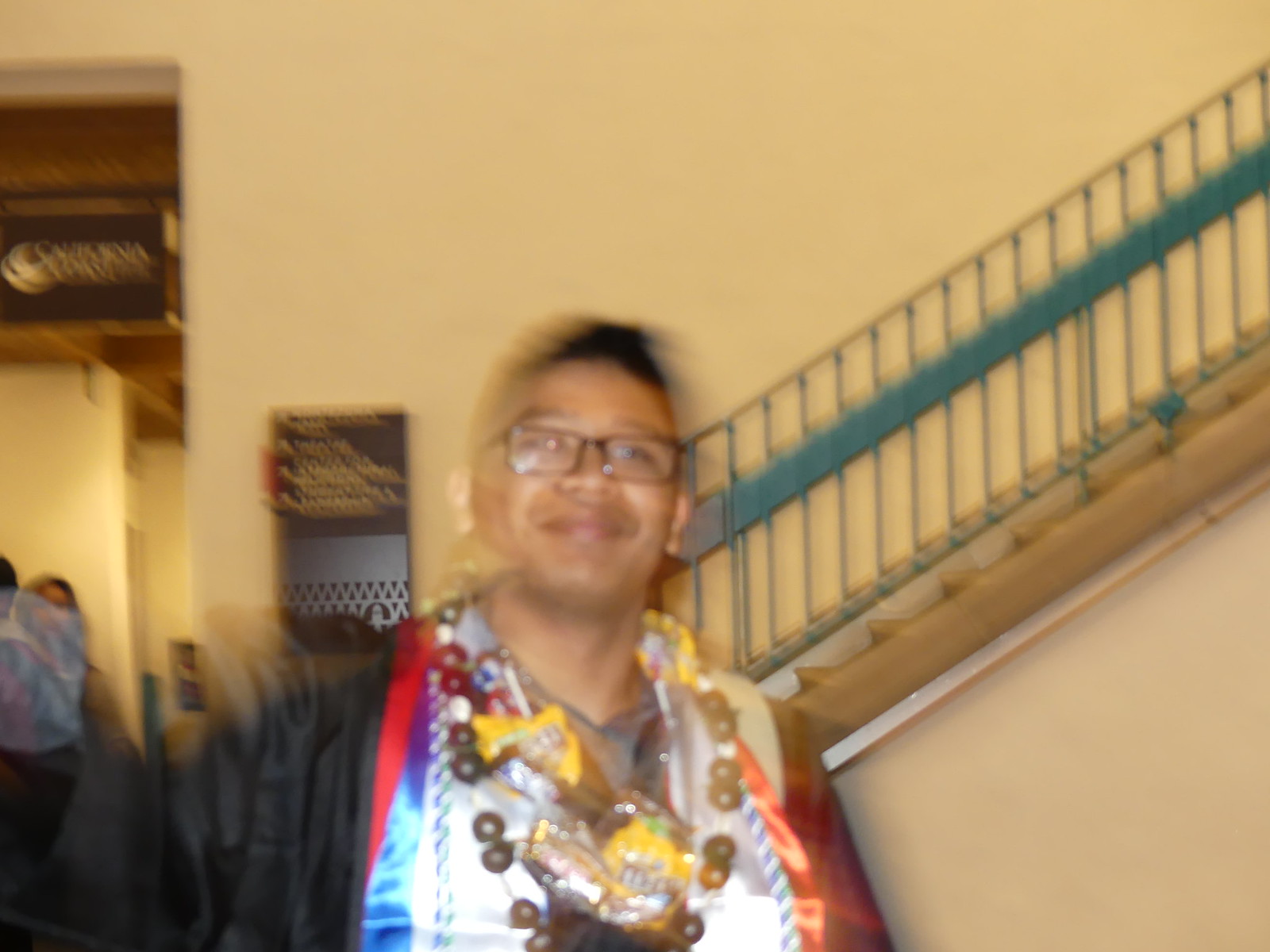In this slightly blurry photograph, a man with short black hair and black glasses is smiling. He is dressed in a black graduation robe, adorned with a red and blue sash. Around his neck is a distinctive black beaded necklace, interspersed with yellow bags of M&Ms. The background features a teal and tan staircase, a white wall, and a black sign with yellow text. Over one of his shoulders, a few people are visible, including an individual wearing a blue shirt and another in a tan shirt.